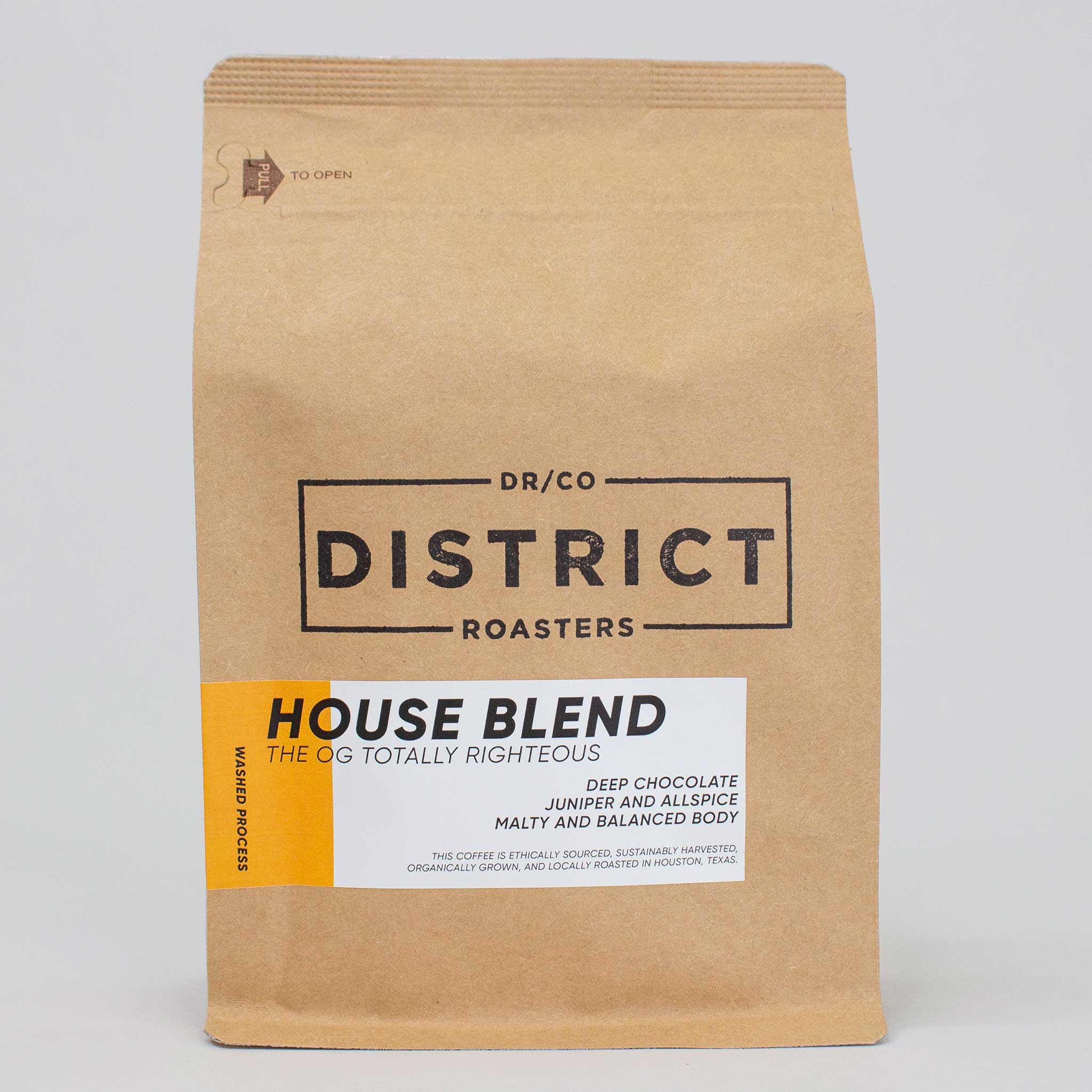The image displays a minimalist, tan cardboard bag of coffee resting on a cream-white background. The bag is sealed at the top, marked with a pull tab and a brown arrow directing "Pull to Open". Prominently in the center is the logo for District Roasters, abbreviated as DR/CO, enclosed in a black border. Below this, in bold black text, it declares the blend as "House Blend, the OG Totally Righteous", accompanied by a detailed description: "deep chocolate, juniper, and allspice, malty and balanced body, washed process." Further emphasizing its quality, the coffee is noted to be "ethically sourced, sustainably harvested, organically grown, and locally roasted in Houston, Texas". A distinctive white and orange label adorns the side, reinforcing the bag's simple yet informative design.